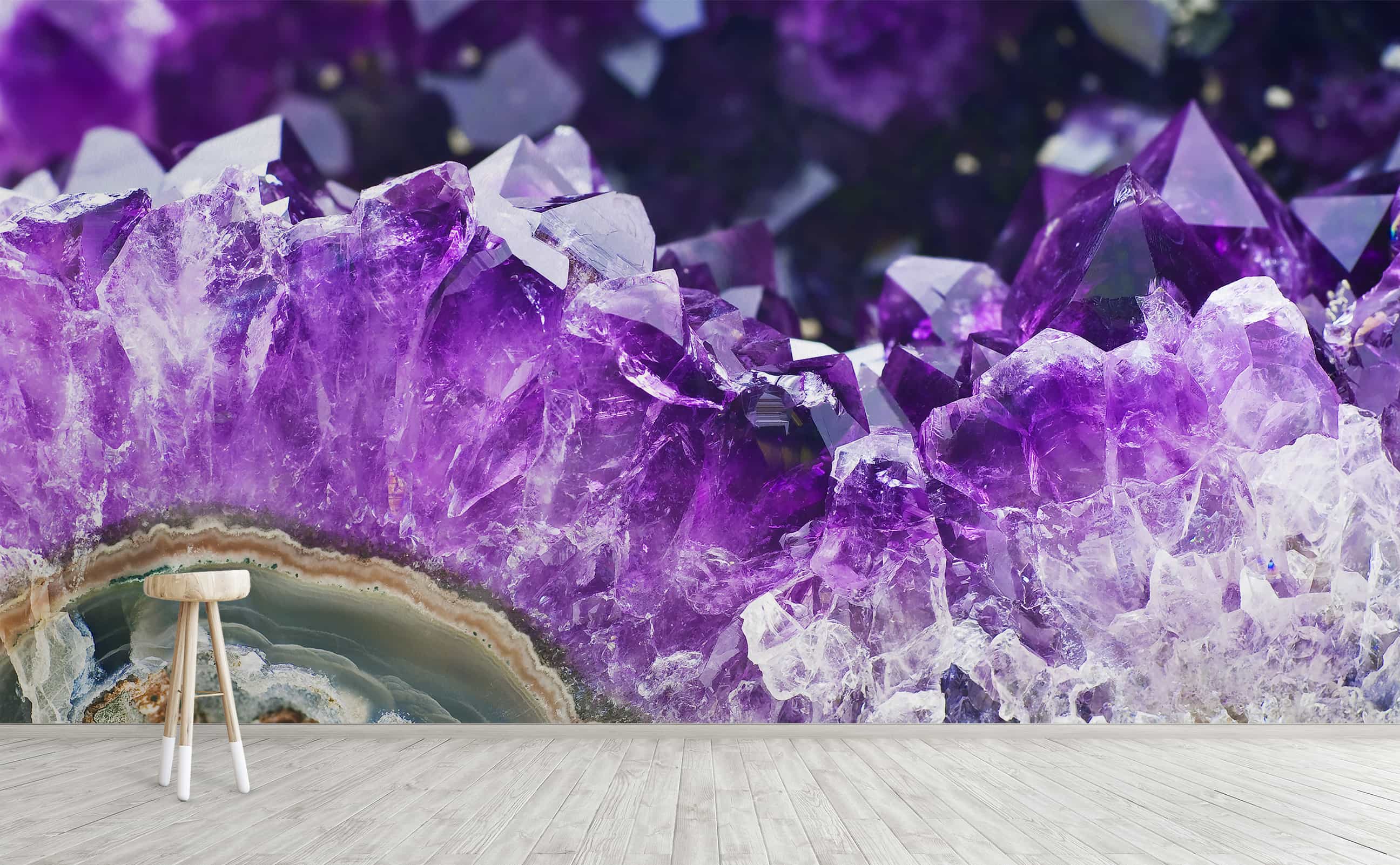The image is a horizontally rectangular, full-color photograph that appears to be carefully staged with artificial lighting. The entire backdrop is a mesmerizing, highly detailed portrayal of a large purple geode. The geode displays various layers ranging from purple amethyst hues to grays, browns, and whites, with clear crystals forming a sparkling cluster in the bottom right corner. The background is filled with more purple geodes and crystals, blurring slightly to enhance the central focus.

The lower portion of the image shows a light gray wooden floor. In the bottom left corner stands a small, natural wood bar stool with three legs, crafted in a tripod shape. The stool's proportions give the appearance that it might be a miniature, adding a unique sense of scale against the enormous, striking geode backdrop. The wooden texture of the floor and the stool complements the earthy tones interspersed within the geode, creating a cohesive and visually appealing composition.